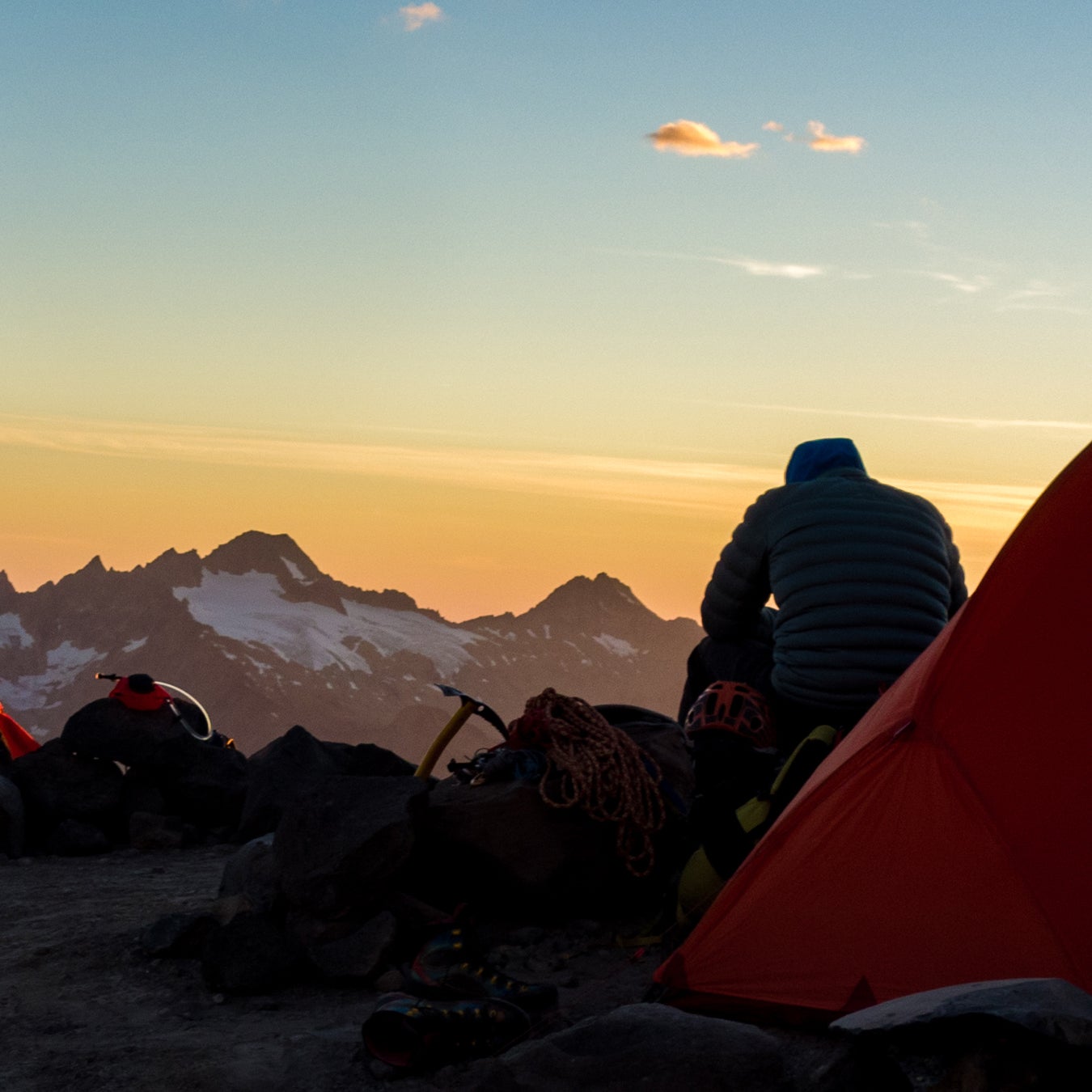The image depicts a serene dawn scene in a snowy mountainous region. The sky transitions from a deep blue to a light orange hue, hinting at the rising sun. A man is seated with his back turned, leaning over with his elbows on his knees, and is dressed in a dark blue parka jacket with the hood pulled up to keep warm. He is positioned beside a red (or pink) tent, partially visible in the bottom right corner of the photograph. Surrounding him is an array of climbing gear, including ropes, backpacks, helmets (one red and black), a pickaxe, and boots. In the background, snow-capped mountains create a majestic silhouette against the sky, completing the tranquil camping scene.